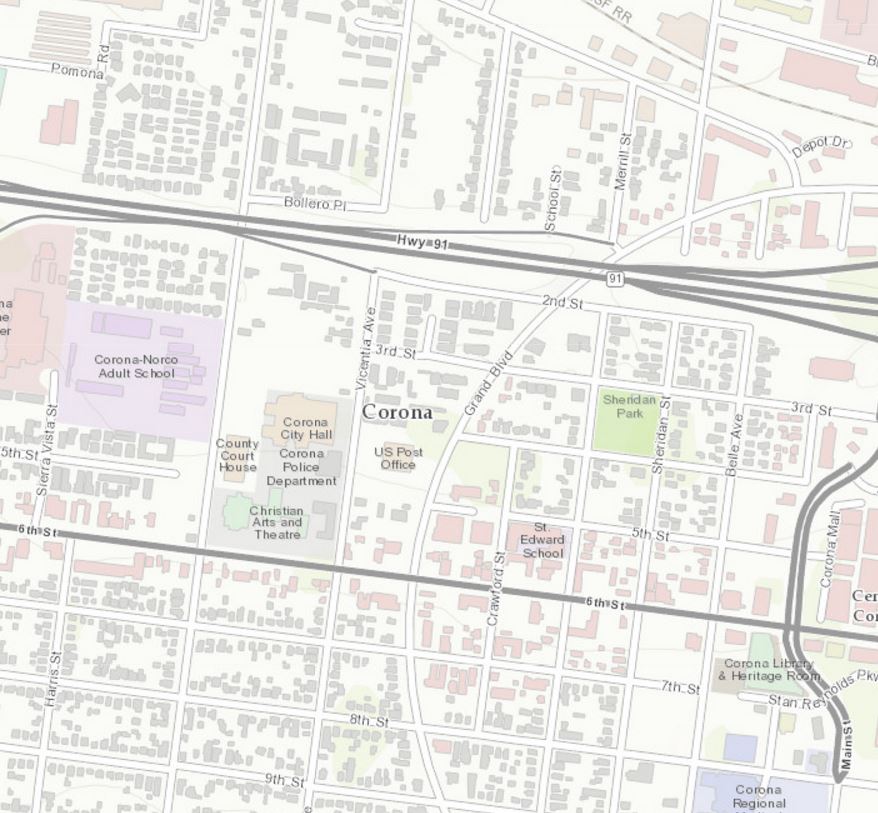This color illustrated map section depicts the city of Corona with a clear and detailed layout. At its core, the map features "Corona" prominently near the center. The typical cartographic lines define the city's infrastructure, including two or three main streets marked by light gray lines which signify the principal roads slicing through the map. Buildings, differentiated in pale gray and pale pink, demarcate various structures that likely denote different types of establishments or zones. Sheridan Park is highlighted with a green shading, indicating a significant recreational area. 

The map's orientation reveals two primary arteries or roads traversing the top and bottom thirds at a slight diagonal from the upper left to the lower right. Within one section, marked in purple, lies the Corona Norco Adult School, underscoring an educational facility of notable size. The Interstate, labeled as Highway 91, provides a major transit route, while 6th Street is identified as a key thoroughfare at the map's lower edge. This map effectively captures a vibrant and structured overview of the cityscape, emphasizing significant locations and infrastructure.